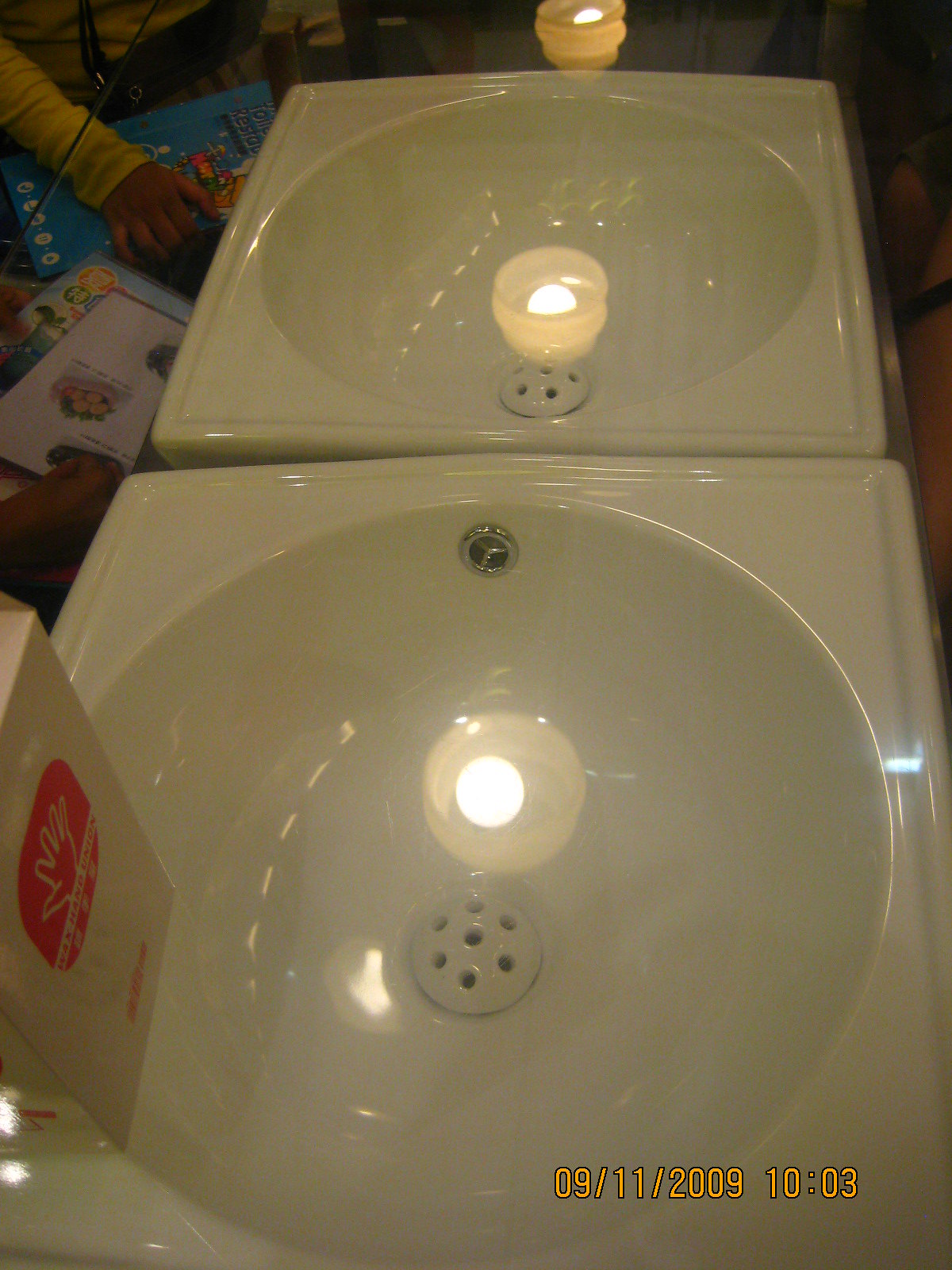The color photo captures a detailed scene featuring two square porcelain-like structures resembling sinks, positioned side by side, on top of a coffee table with a glass surface that reflects overhead lighting. Each structure has a circular bowl in the center with a mound akin to half a golf ball, punctuated with multiple circular holes, serving as a unique design element rather than traditional drains. On the table, adjacent to these structures, a white box with a red logo bearing the word "hand" is visible. In the bottom right corner of the image, a timestamp reads "09-11-2009 10:03."

In the background, to the top left, a child dressed in a yellow long-sleeved shirt can be partly seen, holding a blue book adorned with various colors. Sitting next to the child is another person holding an open book, which seems to display images of vegetables. Scattered around them are multiple children's toys and books, adding a playful and lively touch to the setting.